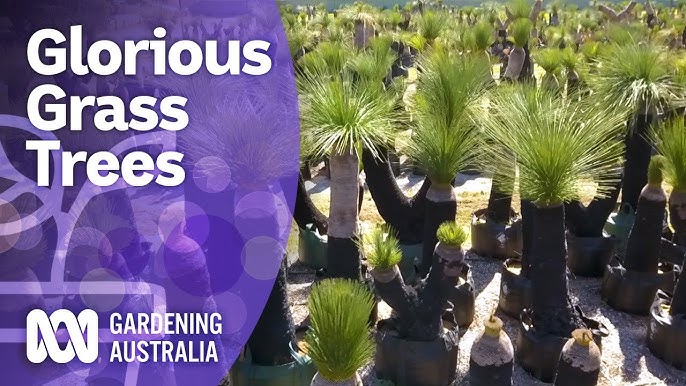The image depicted in the banner promotes a variety of plants and trees available for purchase from a business. The rectangular banner is twice as long as it is tall and is divided into two distinct sections. On the left, a large, semi-curved, semi-transparent purple with varying shades and spots serves as a backdrop for the white text that reads "Glorious Grass Trees." Beneath the text, in the lower-left corner, is the logo and name "Gardening Australia," with the logo featuring a twisted line forming a circle flanked by triangles. The right side of the banner showcases multiple thick trunk trees, identified as the unusual Glorious Grass Trees. These trees feature large, fern-like bushes sprouting from their tops, resembling grass clumps growing out of the trunks. The trees are organized in orderly rows, emphasizing their unique and striking appearance, which is reminiscent of a blend between a palm tree trunk and a dense bush of tall grass.